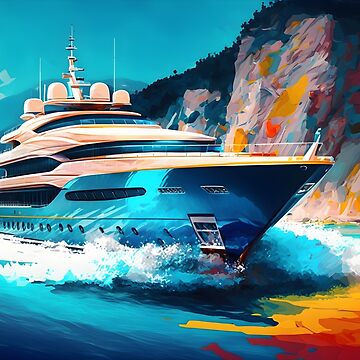This image showcases a beautifully painted depiction of a large, multi-tiered yacht navigating through vibrant ocean waters. The yacht's hull is a striking mix of brushed blue shades, resembling shiny sheet metal, while the upper tiers are beige and white. These upper levels feature rows of windows and a deck with a visible individual and seating arrangements atop. The topmost part of the yacht is equipped with four radar towers and various navigation instruments.

The yacht slices through the teal, foam-capped waves, creating dynamic splashes on either side that add a sense of movement and energy. The water reflects the artist's palette of yellow, orange, and red hues, which are concentrated in the bottom right corner of the scene. These vivid colors also appear on the multicolored cliffs to the right, with predominant gray tones interspersed with patches of orange and red, and greenery crowning the tops of the cliffs.

In the background, a cyan sky stretches above a distant mountain range, adding depth and a sense of vastness to the composition. Overall, this painting captures a moment during the day where natural beauty and human craftsmanship converge in a breathtaking maritime scene.